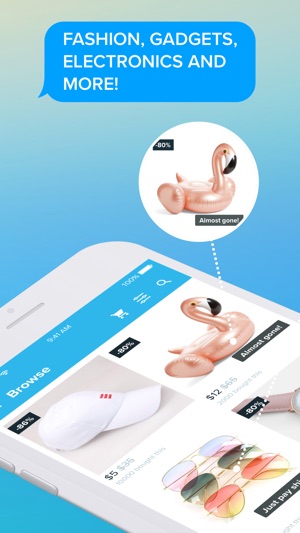A detailed screenshot preview of a shopping app, as seen in the Apple App Store, is featured. The image simulates the interface of the app, designed for an iPhone, which is showcased at an angle. The background gradient transitions from a greenish hue at the top to a solid blue at the bottom. At the top of the screenshot, a speech bubble with a blue background and a pointer adds emphasis with the text: "Fastening gadget, electronics, and more!" in three lines, suggesting excitement and variety in the offerings.

In the main part of the screenshot, you can see a partially visible iPhone screen displaying the shopping app's user interface. The app showcases an assortment of items available for purchase, arranged in a grid format. On the top row, the app depicts several purchasable products, including a hat, what appears to be a swan-shaped float, sunglasses, and another indistinct item. The swan float is particularly highlighted, accentuated with a white dotted line leading to a circle above it, drawing attention to this specific product as a featured item.